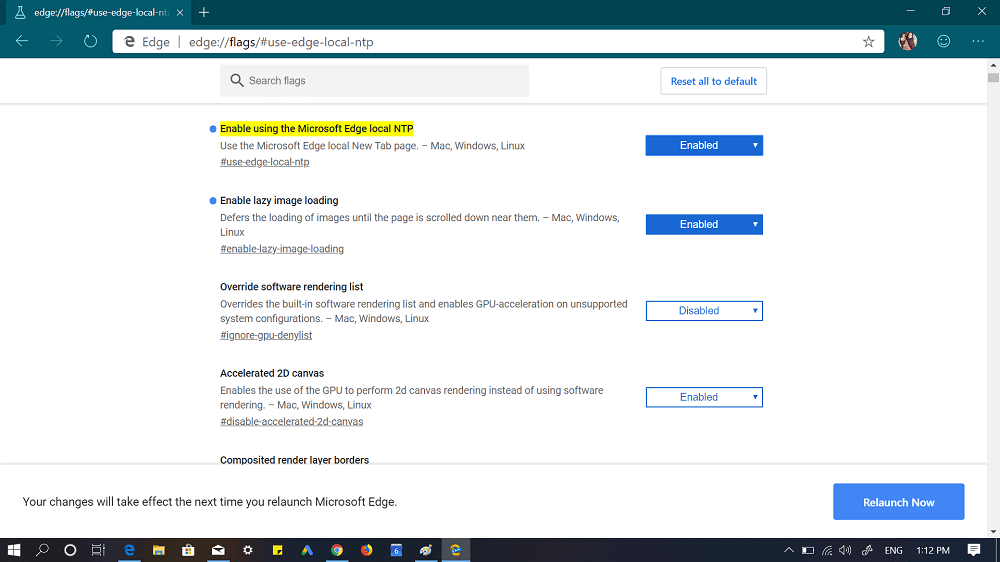This image captures a close-up view of a Microsoft Edge browser window with a plethora of technical settings visible. The tab is labeled "Edge Flags" and prominently displays the subheading "Use Edge Local." The screen appears blurry even at a zoom level of 200%, making the text challenging to read. In the search bar within the settings, the term "Search Flags" is displayed, though no active search query is present. All the settings are set to their default states.

The first noticeable setting is "Enable Using the Microsoft Edge Local NTP," which is highlighted with a blue dot indicating it is toggled on. Below this, the "Enable Lazy Image Loading" option appears, described as a feature that defers image loading until the user scrolls near them. This setting is applicable to Mac, Windows, and Linux systems.

Further down, the image shows options to "Override Software Rendering List" and "Accelerated 2D Canvas," followed by "Composited Render Layer Borders." At the bottom of this list, a message indicates that any changes made will be implemented the next time Microsoft Edge is relaunched, accompanied by a "Relaunch Now" button to prompt immediate restart of the browser.